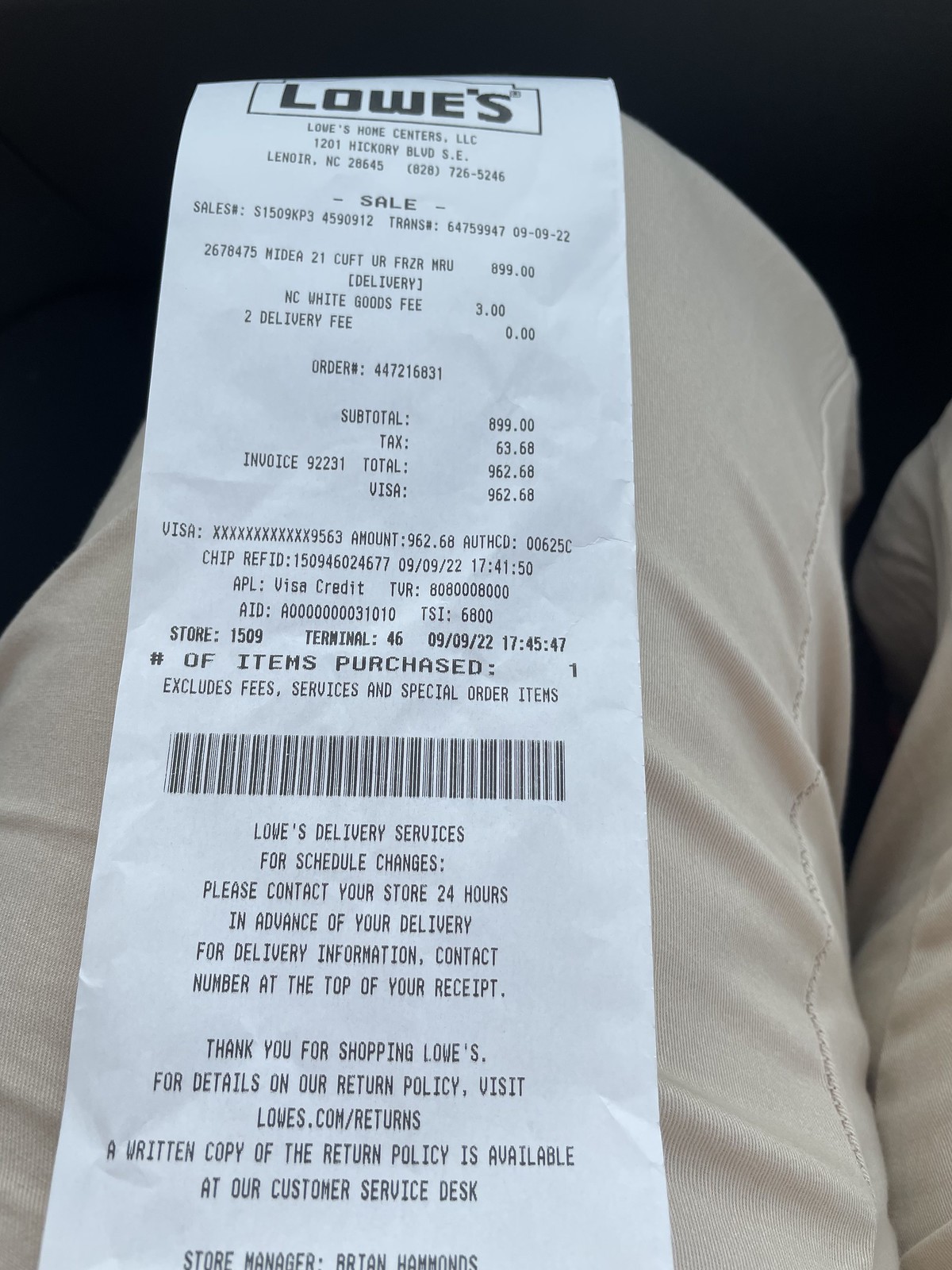In the dimly lit confines of what appears to be a car's footwell, a photo captures someone’s legs in light tan pants. Most prominently displayed on the left leg, partially obscured by shadows, is a long, white, rectangular receipt from Lowe's. The receipt details a significant purchase for a total of $962.68, charged to a Visa card. The purchased item is partially readable as a "21 cubic foot" appliance, possibly a freezer. Below the transaction details, the receipt includes instructions regarding Lowe's Delivery Services and store contact information for scheduling changes, as well as a return policy blurb. The store manager's name, Brian Hammonds, is listed at the bottom. The background surrounding the legs is very dark, suggesting that the photo was taken inside a vehicle.